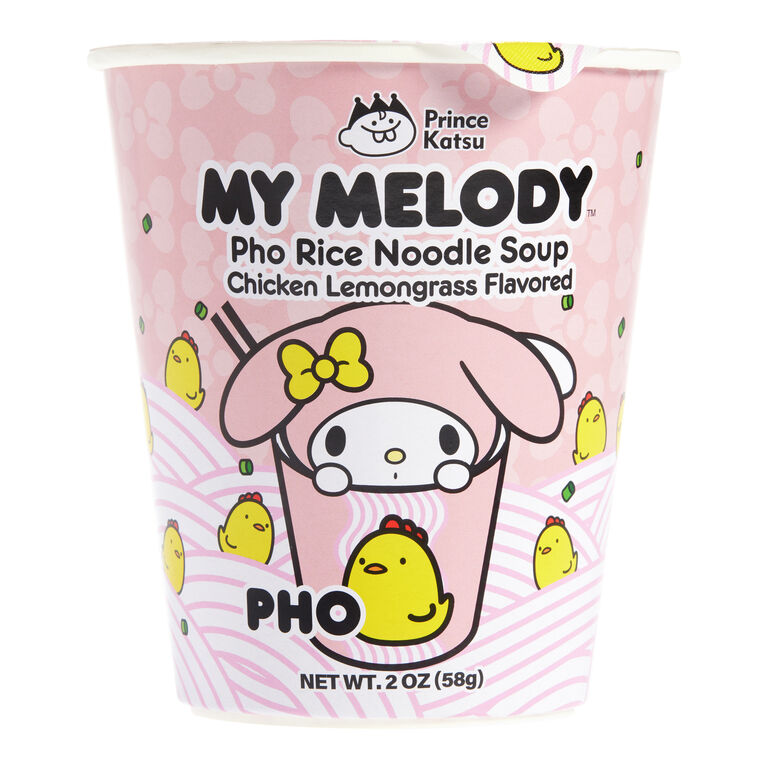This is a highly detailed photo of a food product—a cup of noodles—with a predominantly pink and white design. The brand, Prince Katsu, prominently features text that reads "My Melody Pho Rice Noodle Soup, Chicken Lemongrass Flavored," with the net weight clearly stated as 2 ounces (58 grams). The cup is adorned with charming, childlike imagery: a central cartoon character, resembling a rabbit with drooped ears, peeks over the edge of a cup within the illustration. This character has black eyes, a yellow nose, and a yellow bow on its head. Scattered across the cup are multiple small, yellow chicks, each with a red comb. The bottom of the cup showcases white and pink stripes, adding to the playful aesthetic.